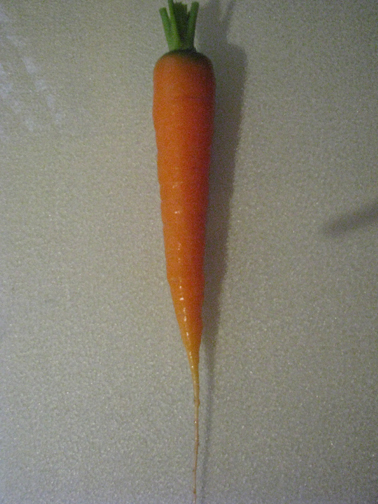This is a detailed photograph of a freshly picked, full-size carrot, captured vertically in a small rectangular frame. The vibrant orange carrot, lying on a speckled grayish kitchen countertop, appears damp with a few dirt smudges and a distinctive long, slightly crooked, root extending out of the bottom of the frame. At the top of the carrot, you can see remnants of green stems, now cut short, and a slightly darker area indicating where the carrot might have been exposed above the soil. The image is centered, with the carrot casting a shadow on the textured white surface beneath, illuminated by a strong light source from above.